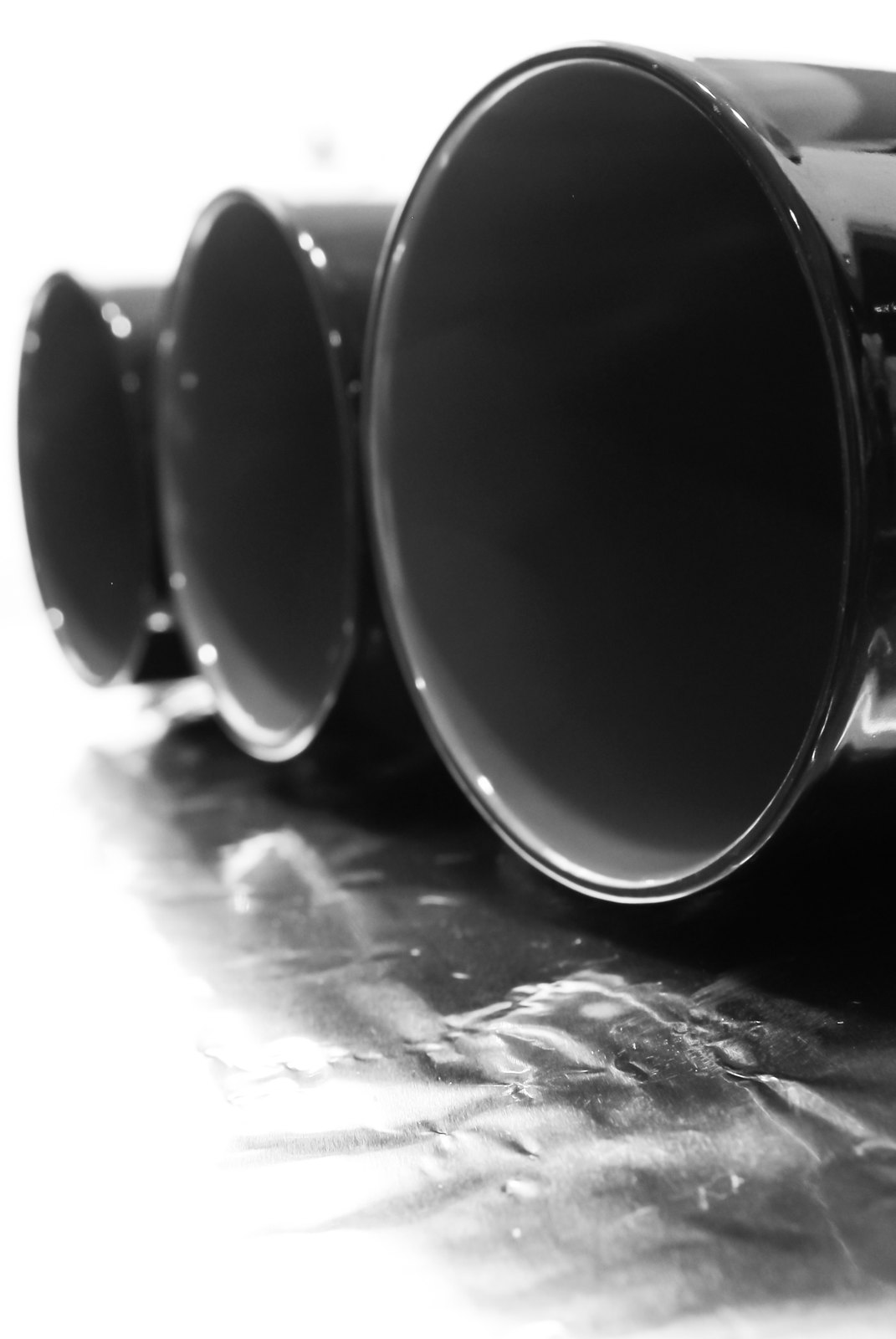In this simple and striking black and white photograph, three round, dark cylinders, resembling coffee cups, lie on their sides atop a crinkled layer of tinfoil. The largest cup, positioned prominently at the right forefront, catches the viewer's eye first, while the other two, appearing progressively smaller, extend toward the left. The exterior of the cups is a smooth, shiny black, while their interiors, filled with shadow, reveal a lighter gray hue, creating a striking contrast. The tinfoil below them is marked with indentations and wet spots, adding texture and depth to the scene. Despite their alignment, the rims of the cups do not touch the foil, and the overall effect is of a minimalist composition with a washed-out background around the foil.